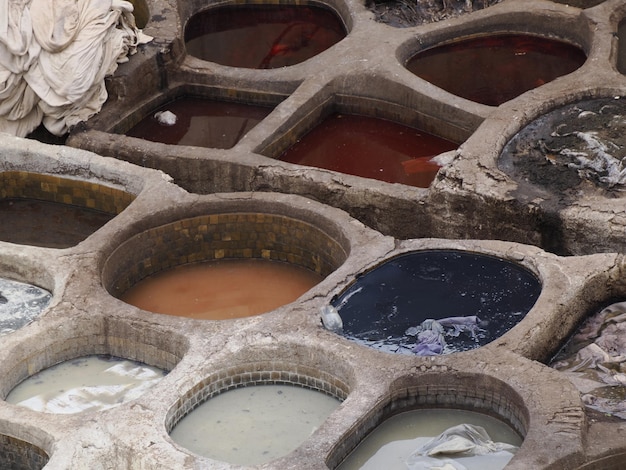The image depicts a sprawling, stone structure resembling a prehistoric or medieval bath complex. The baths are irregularly shaped and interconnected by stone walls, which divide them into distinct sections. Each pool is lined with square mosaic tiles and contains liquids of varying colors. In the back of the image, there are two circular pools filled with a brown liquid, while in front of them are two square pools; the left one has a brown liquid, and the right one contains a striking red liquid. A higher, shallower pool nearby holds a dark liquid with white swirls, offsetting the earth tones. Moving to the front rows, there is a square pool with brown liquid, a circular pool with light brown or tan liquid, and another circular pool with dark blue liquid. The pools in the frontmost row feature various shades of white, predominantly rounded in shape. Additionally, a sculpture resembling a giant flower, made of stone, is partially visible in the back left corner of the image, adding to the elaborate and ancient aesthetic of the scene.